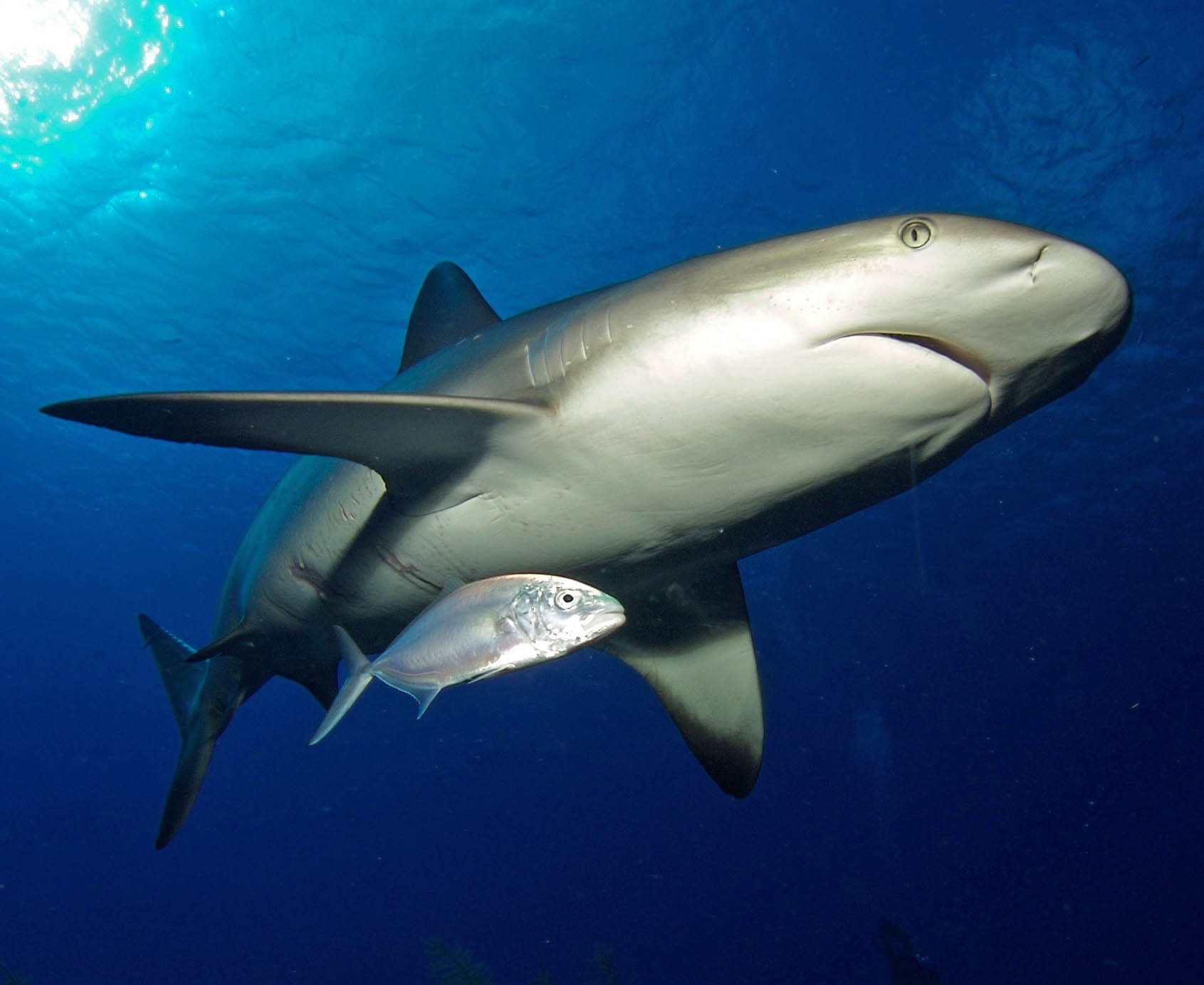This underwater photograph captures a serene scene in the crystal-clear, deep blue ocean. Dominating the frame is a shark, viewed from below, with its lighter gray underside and darker gray top, accented by numerous scars trailing down its torso. Its mouth is closed, and distinct gray eyes, with small black slits, are visible. Directly beneath its belly, a smaller, gray fish with similar gray eyes glides effortlessly. The fins of both sea creatures are extended, giving the impression of smooth, synchronized movement. The shark and the fish both swim from the left to the right side of the image. The top left corner of the photograph features rays of sunlight piercing through the water. Neither the shark nor the fish seem to be aware of each other, gliding peacefully in the clear, tranquil ocean.